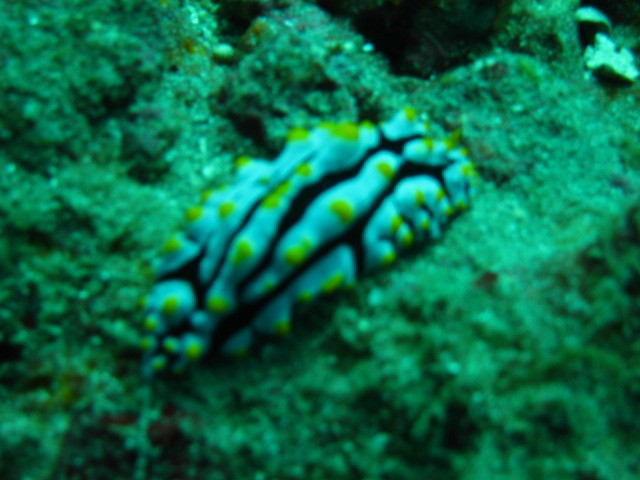The photograph captures a mysterious, vibrant creature, likely underwater, resting on a mossy, rock-like structure. The setting suggests an aquarium due to the lighting and composition. The creature boasts a cylindrical, slug-like shape adorned with puffy, light blue and black stripes. Lime green and yellowish raised dots punctuate the blue areas, adding to its vivid appearance. Although the image is slightly blurry, suggesting it wasn't taken professionally, the rich colors and intricate details of the creature are striking. The backdrop features a mossy, emerald green texture, which enhances the underwater ambiance and the enigmatic allure of the creature, possibly an unknown marine animal or plant life.